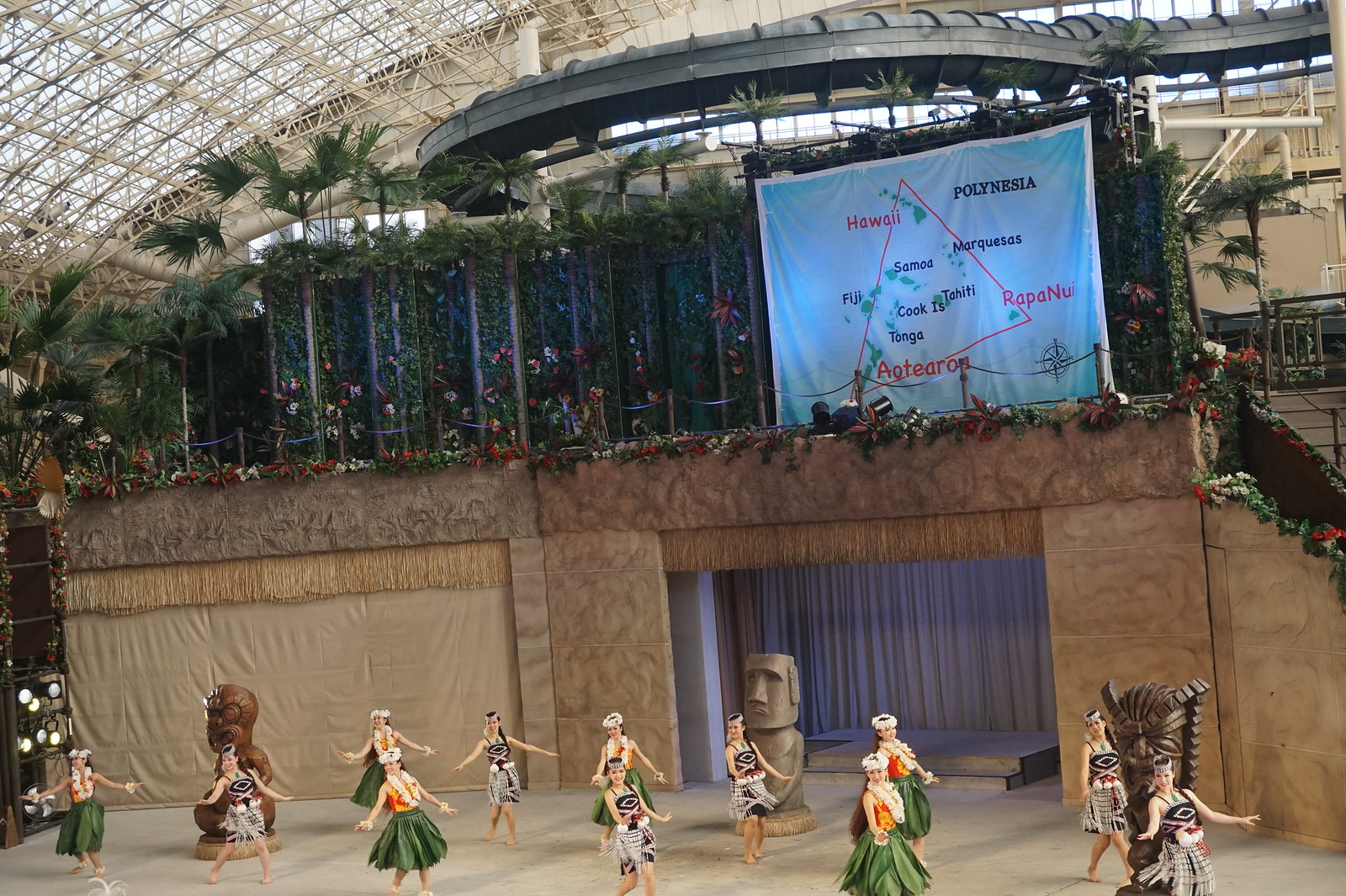The image depicts a lively event taking place on a large, elevated indoor-outdoor stage with a latticework metal roof, which gives the venue an open, island-like atmosphere. The floor appears to be concrete, and the backdrop features a combination of brown curtains and flowered effects, with tiki statues adding to the Polynesian theme. At the center of the stage, a blue banner highlights different parts of Polynesia, including Hawaii, the Cook Islands, Tonga, and Fiji, forming a triangular display.

On stage, a group of performers are engaging in a traditional dance. They are clad in vibrant costumes: some women wear green grass skirts, sleeveless orange tops, leis, and decorative headpieces, while others are dressed in black and white traditional attire. All dancers have black hair and are poised with their arms extended, deeply immersed in their choreography. In the background, a gray stone tiki statue can be seen, enhancing the cultural authenticity of the scene. This dynamic performance and detailed setting combine to evoke the festive spirit of a Hawaiian luau.